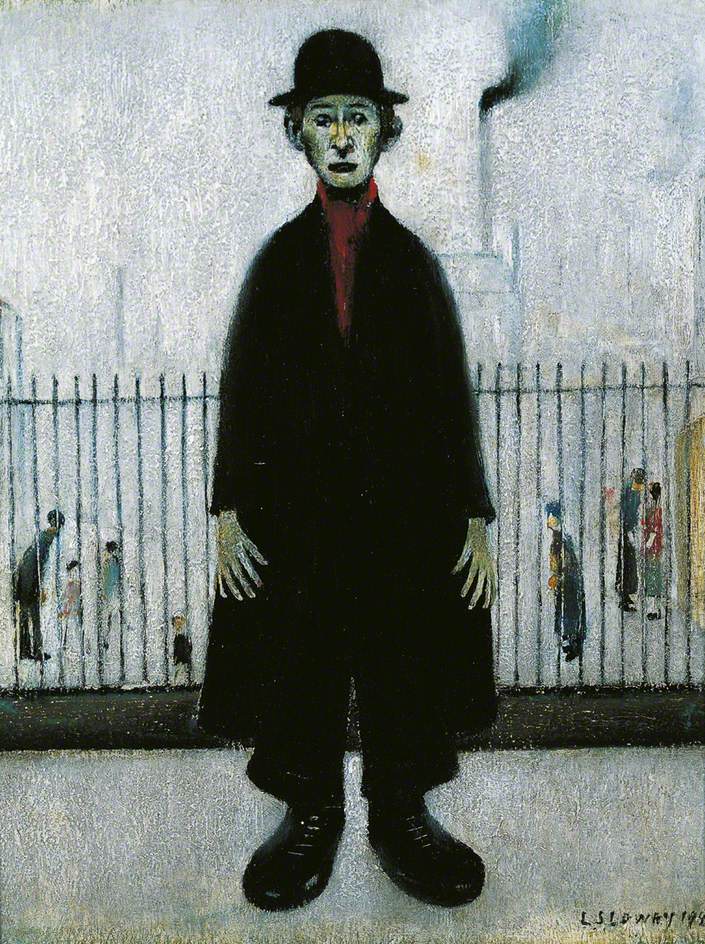This painting, titled "A Lancashire Cotton Worker" by L. S. Lowry, created in 1944, depicts a poignant scene in portrait orientation. The central figure is an adult male standing on a gray concrete surface, facing the viewer with a sad, almost spooked expression. Dressed in a long black overcoat, black pants, and oversized black boots, his attire is complemented by a black hat that gives him a semblance of Charlie Chaplin, albeit without the mustache. His skin appears bluish-gray, and he wears a red garment—either a scarf or part of a turtleneck sweater—under his coat.

The man's exaggerated physical features include super large hands and feet, depicted in a manner characteristic of naive art, specifically primitivism. His eyes appear closed, adding to his melancholic demeanor. Behind him is a black metal railing type fence, beyond which several blurred figures of adults and children mill about, immersed in indistinct conversations. The background further recedes into a gray to white fog, with the faint silhouette of a house featuring a long chimney with smoke trailing into the mist. The overall palette is muted, with dominant shades of black, gray, and white, enhancing the sense of solemnity and industrial melancholy.